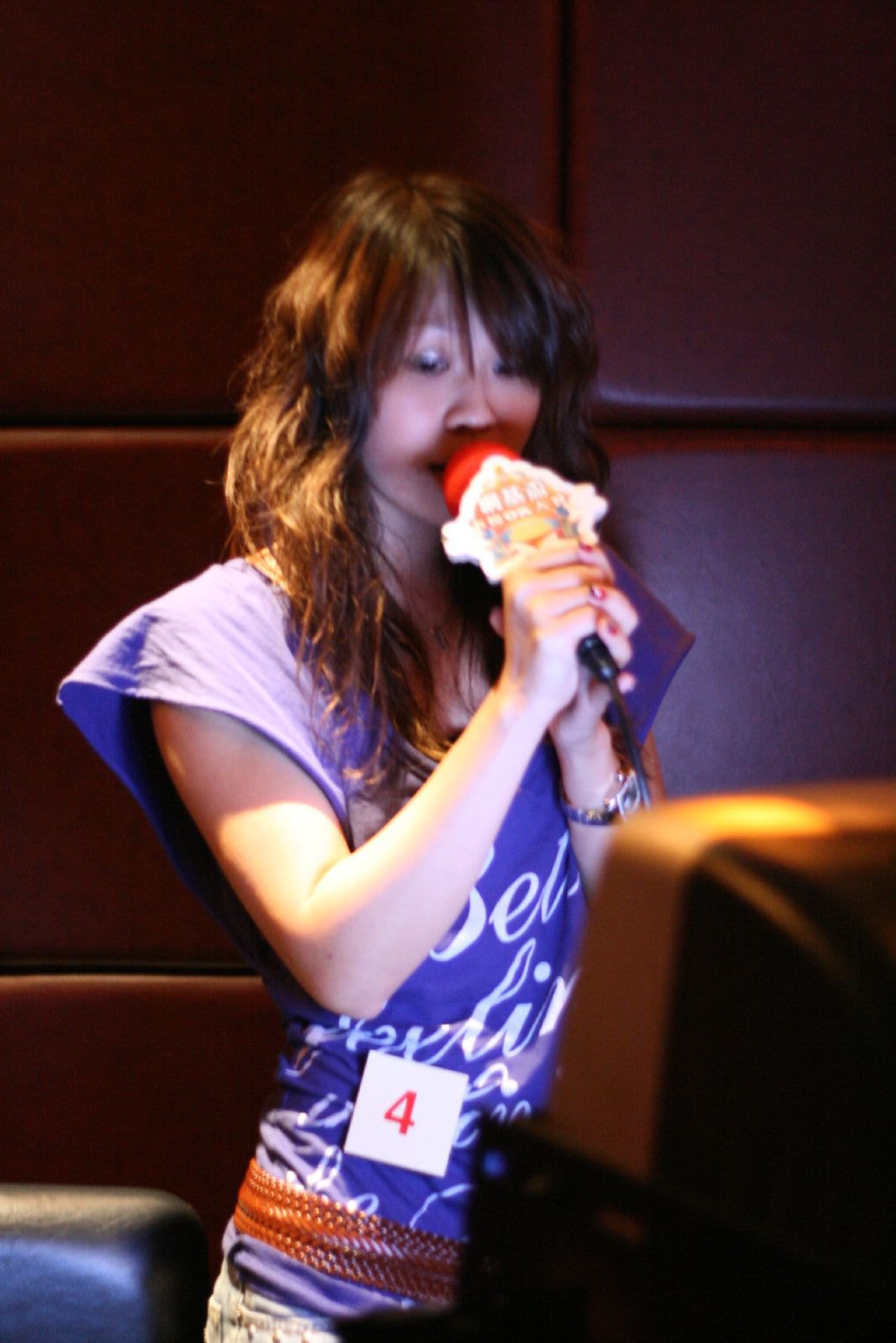In the image, an Asian woman with slightly wavy dark hair styled in bangs is holding a microphone with a red screen guard. She appears to be singing or giving a speech, possibly at a karaoke event, as she's looking at a monitor, likely displaying lyrics. The woman is dressed in a purple top with white cursive writing and a brown belt around her waist. She also has a square white sticker on her shirt with the red number 4, indicating she might be contestant number 4. Her eyeshadow appears to be shiny, and the ambient lighting in the room is orange-ish and dark, with brown, padded cushion-texture walls. Sunlight streams in, illuminating her arm and hair, adding a warm touch to the scene. There's a TV visible in the right corner of the image, showing only its back, further suggesting she is looking at it for lyrics or prompts.